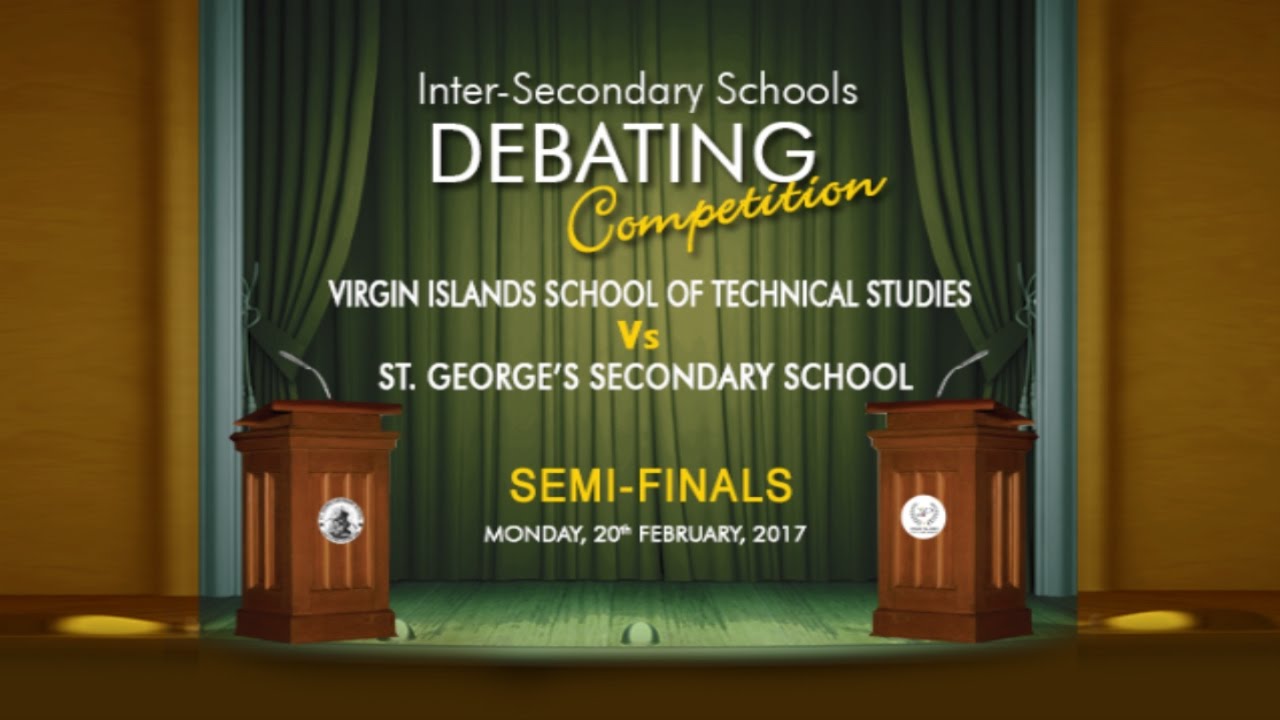The image is an advertisement for the Inter-Secondary Schools Debating Competition. It portrays a detailed setup of a stage setting, highlighting the semifinals between Virgin Islands School of Technical Studies and St. George's Secondary School scheduled for Monday, the 20th of February, 2017. Dominating the background is a deep forest green curtain with light blue accents, set against a gold-colored wall. The green curtain serves as the backdrop for white and yellow text announcing the competition details. Flanking the stage are two debate podiums, positioned on the left and right, each in brown wood with a distinctive white seal in the center. The floor appears to be a greenish wooden color, complemented by wooden elements on either side of the stage and a blue wooden frame around it. The bottom part of the image shows a brown section of the building, grounding the entire stage setup in what seems to be a theater.